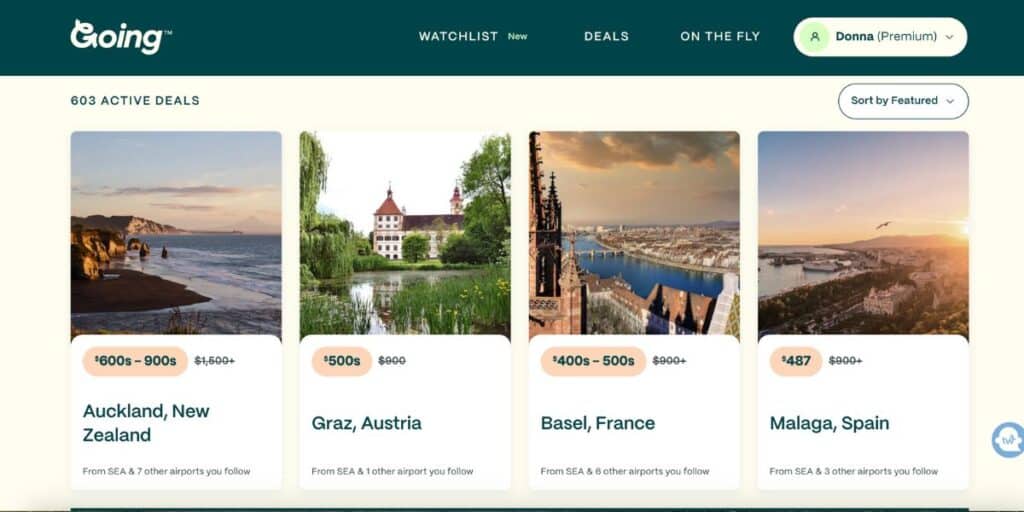Screenshot from a travel website interface:

In the upper left-hand corner of the screenshot, the website logo reads "Going," with the letter 'G' creatively designed to resemble an arrow. Below the logo, the website lists "603 active deals." 

Centralized at the top, several options are displayed in the navigation bar: "Watch List" (labeled as 'new'), "Deals," "On the Fly," followed by the user's name "Donna" with "premium" in parentheses, indicating a premium membership or account.

On the right side, a dropdown menu option "Sort by featured" is visible, implying the user can sort deals by featured listings.

Four travel deal options are showcased from left to right:

1. The first deal lists a range of $600 to $900, with a previous higher price of $1,500 crossed out. The destination highlighted is Auckland, New Zealand.

2. The second deal offers a price of $500, down from a previously listed $900, with the destination being Graz, Austria.

3. The third deal ranges from $400 through $500, with a $900+ original price crossed out. The destination for this deal is Basel, France.

4. The fourth and final deal shows a price of $487, reduced from over $900, offering a trip to Malaga, Spain.

Each option highlights significant savings, showcasing drastic cuts from their original price, offering compelling discounts for potential travelers.